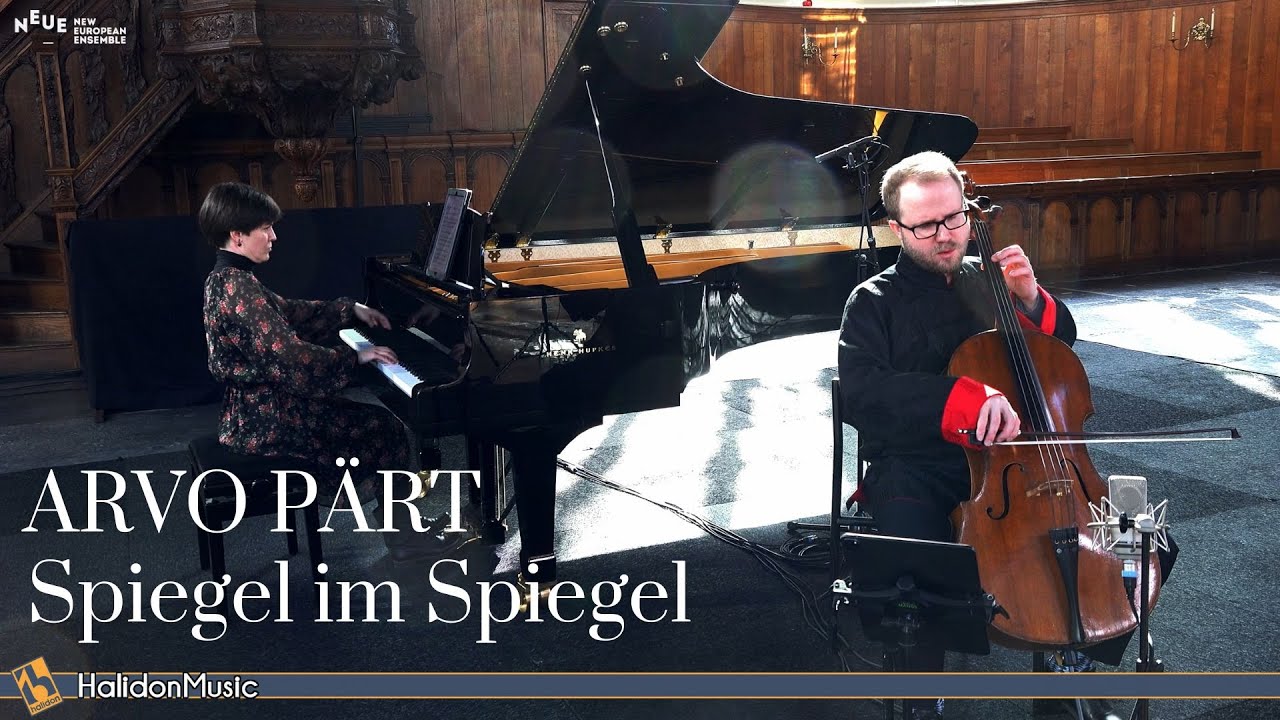The image depicts a professional musical performance, likely captured for an advertisement. At the forefront stands a male cellist, identifiable by his glasses and black attire accented with red cuffs. He is positioned in front of a microphone, indicating a possible recording session. Adjacent to him is a female pianist with short black hair, seated at a grand black piano, with the lid open. The performance setting is visually warm with a wooden backdrop and stone flooring, suggesting an intimate stage or a finely designed room. In the background, to the left, the poster text reads “Ärvo Pärt Spiegel im Spiegel,” with the 'A' bearing an umlaut, hinting at German or Austrian origins. Below this, “Halidon Music” is written alongside an orange and blue logo featuring a musical note. Light illuminates the scene, creating a bright and inviting atmosphere under the piano.